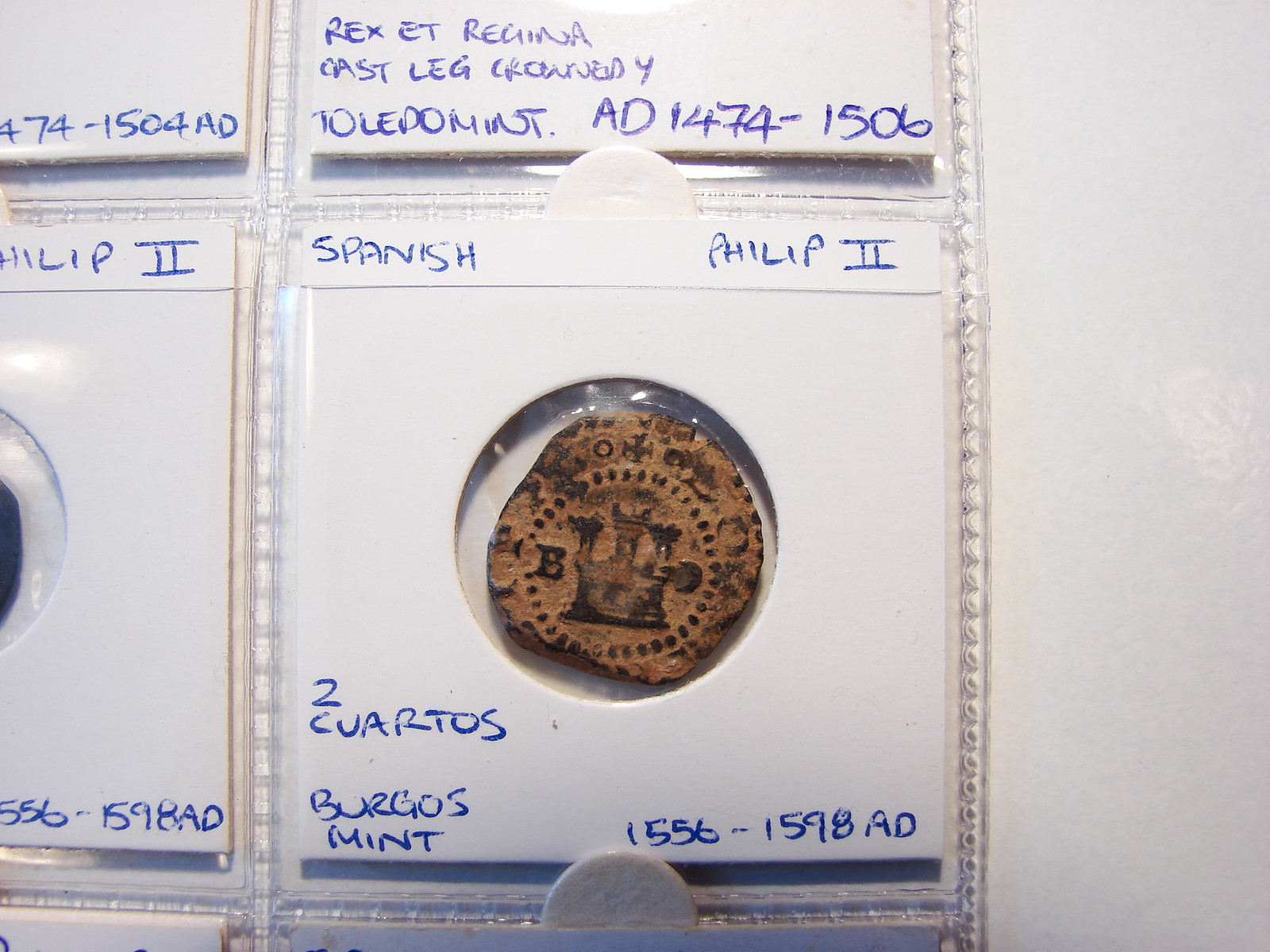This photograph showcases a detailed coin collection album, with the spotlight on a specific Spanish coin from the reign of Philip II. Encased in a white plastic holder with clear covering, the coin is prominently positioned at the center of the holder. The label at the top left reads "Spanish," and "Philip II" is noted at the top right, both inscribed in blue ink. Below the coin, inscriptions detail its value as "Two Cuartos," minted in Burgos, with its age noted as 1556 to 1598 A.D. The coin itself appears to be crafted from a reddish-brown material and features an emblem of a castle in its design. The coin displays considerable wear, suggesting it may never have been perfectly round. Surrounding the highlighted coin, parts of other coin holders are visible, indicating this is part of a larger collection page.